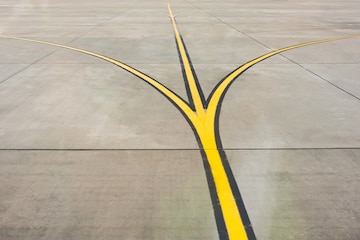The image depicts a minimalist piece of art on what appears to be a concrete ground, characterized by multiple brownish-gray slabs with visible joints running vertically. The background, divided by a faint gray line that stretches from the bottom right toward the center left, is slightly darker at the bottom compared to the top, suggesting a tan wall area. Prominently featured in the artwork is a black-outlined, three-pronged design painted in school bus yellow. This design, with two outer prongs branching off to the left and right and a central prong extending upward, somewhat resembles a chicken's foot or a devil's pitchfork. The entire image is clean and devoid of labels or additional scenery, emphasizing the stark, abstract nature of the mural that extends off the page on all sides.